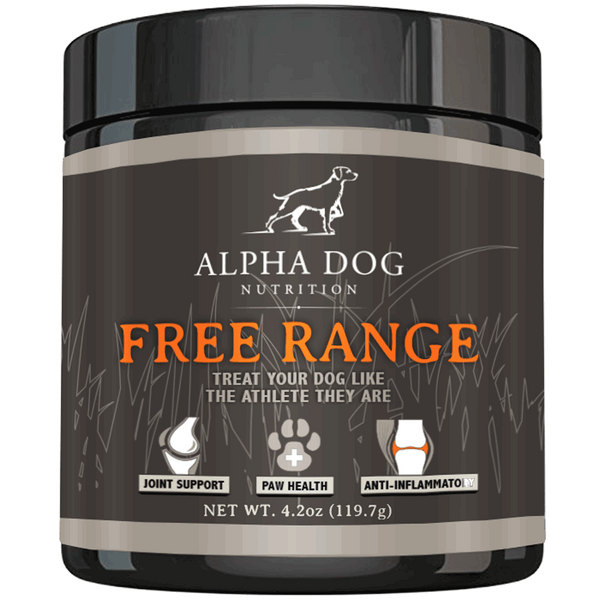The image shows a short, thick jar with a black screw-top lid, containing a dark chocolate brown dog supplement branded as Alpha Dog Nutrition. The label prominently features a detailed drawing of a white spaniel with a brown body, poised with its leg up, suggesting it's eyeing a bird. The depicted dog is near the top of the label. The brand name "Alpha Dog Nutrition" appears beneath the dog image, in white letters. The product name "Free Range" is highlighted in bright orange letters, followed by the tagline "Treat Your Dog Like the Athlete They Are" written in white. The label also includes three small, detailed images: a knee joint labeled "Joint Support," a dog's paw with a white cross tagged "Paw Health," and another knee joint titled "Anti-Inflammatory." At the bottom, the label indicates the net weight as 4.2 ounces (119.7 grams), alongside a tan line encircling the base of the container.